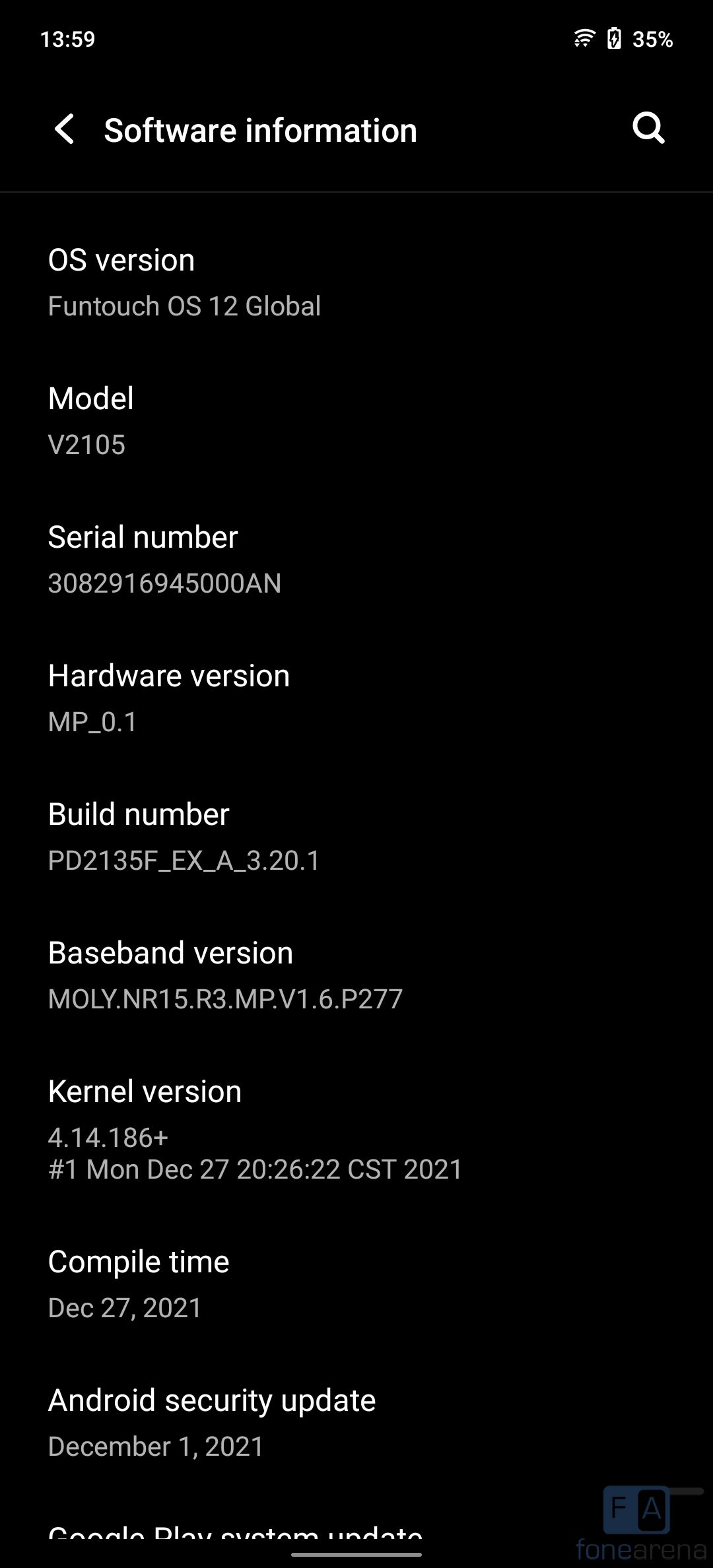A detailed screenshot of a phone displaying its Software Information menu in Night Mode. The dark background contrasts with the white text for easy readability. The top of the screen features a magnifying glass icon, indicating a search option within this menu. 

Key details shown include:
- OS Version: FunTouch OS 12 Global
- Phone Model: V2105
- Serial Number: 3082916945000AN
- Hardware Version: MP Lower 0.1
- Build Number: PD2135_EX_A_3.20.1
- Standard Version: MOLY.NR15.R3.MP.V1.6.P277
- Kernel Version: 4.14.186+
- Build Date: Monday, December 27, 2021, at 8:26 PM Central Standard Time (CST)
- Android Security Update: December 1, 2021

This snapshot encapsulates comprehensive technical data, essential for troubleshooting, verifying updates, or understanding the software environment of the device.